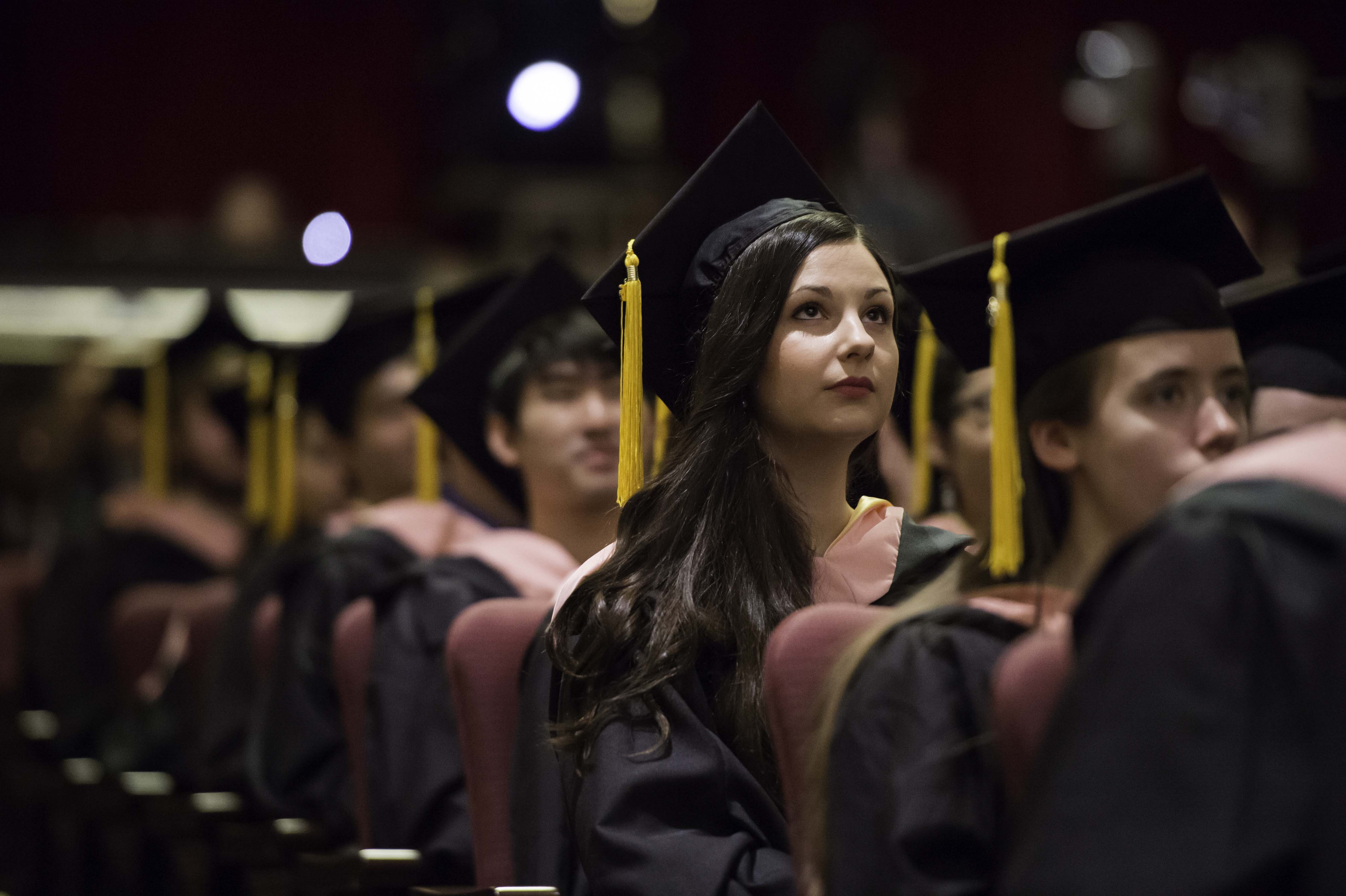In a realistic, horizontally oriented photograph of a graduation ceremony, a sea of graduates dressed in black robes and caps with yellow tassels is seated in mauve-colored chairs. The graduates, likely teens or in their early 20s, wear pink stoles over their gowns. The backdrop consists of black with softly glowing white lights, slightly out of focus. At the center right of the image, a young woman with fair skin, dark hair, and striking dark red lips stands out as the focal point. She gazes upward with her brown eyes, possibly towards a speaker or the stage. An Asian man is seated behind her, while a girl with brown hair is visible in front. Though the other attendees fade into a blur, the sense of shared anticipation for the graduation stage unites the scene.